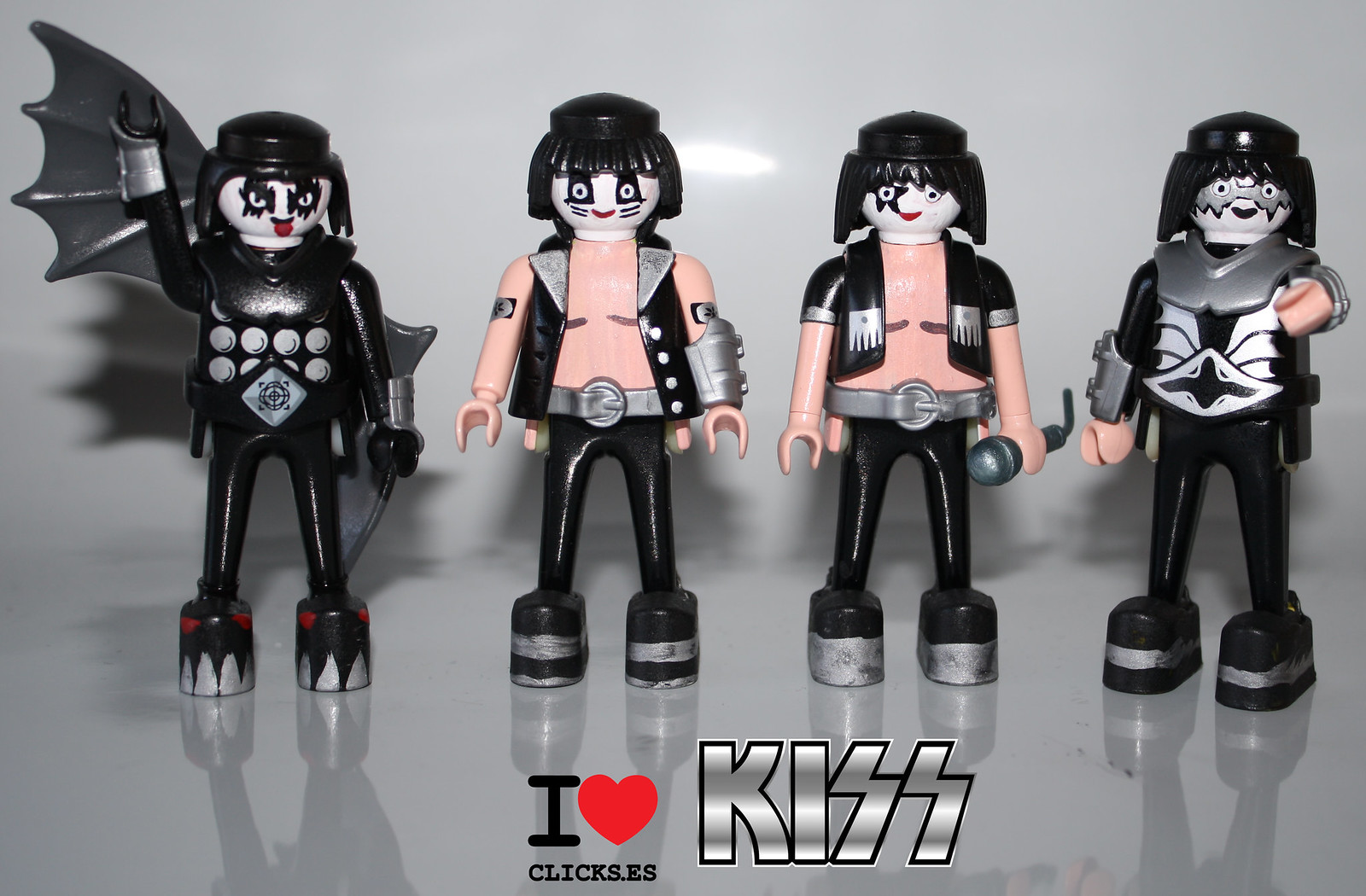This image showcases a collection of four miniature dolls designed to resemble LEGO figures, each meticulously painted to emulate the iconic rock band KISS. The dolls stand upright on a glossy white surface. At the bottom of the image, text reads "I ♥ CLICKS.ES" alongside the KISS logo in silver letters, enhancing the photo's digital, promotional feel.

The dolls are dressed in classic KISS attire, sporting distinctive face paint and long hair. The first doll on the left features white face paint with jagged black bat wings around its eyes, complete with a bat wing accessory on its back, a raised arm, and platform shoes. The second doll is smiling and painted to resemble a cat, wearing a vest over a bare torso and also in platform shoes. The third doll has an open shirt with a star over one eye. The final doll appears to be decked out in metal armor, including a helmet-like face shield pattern. The dolls exhibit various poses, with one holding a stick-like accessory, another with a microphone, and another pointing, effectively capturing the unique personas of the KISS band members.